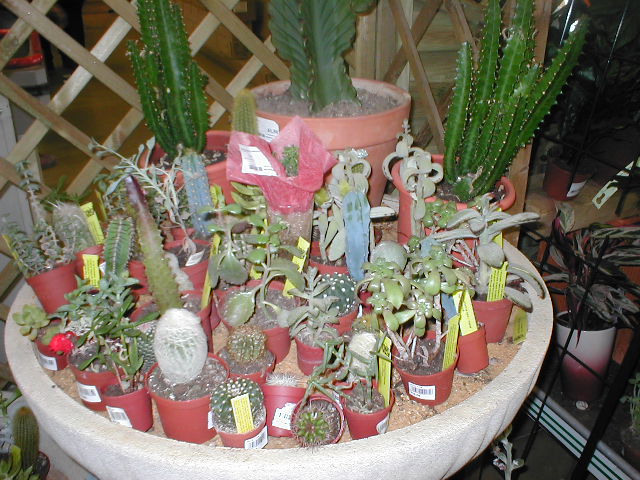In the center of the image is a large, round concrete dish that resembles a birdbath, filled with decorative dirt or sand. This planter holds a variety of cacti and succulents, each in its own small, red flower pot. The cacti range in size and type, with taller, slender varieties towards the back and shorter, rounder ones in the front. All plants are green, although some may have a touch of red, and each pot has a yellow tag and a sticker barcode. The dish is slightly positioned to the left, occupying a significant portion of the white table it rests upon. Also visible in the background to the right is an additional plant stand with more plants, adding to the impression that this setup might be a display for sale. The photograph is taken from a front view, capturing the intricate details and diverse forms of the cacti.